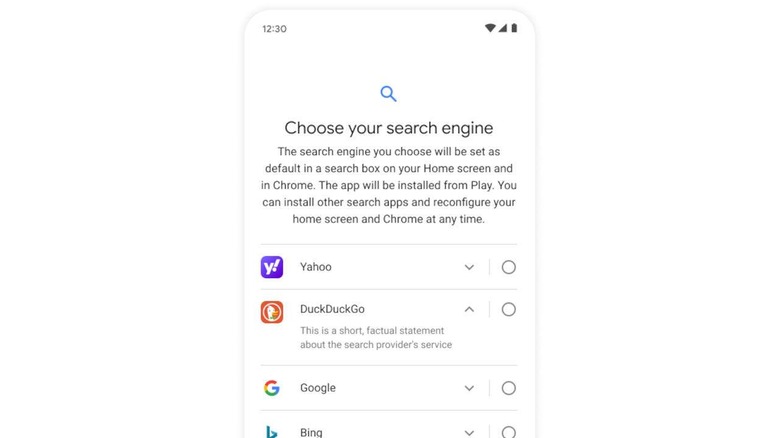This smartphone screen displays a setup interface for choosing a default search engine. At the top left of the screen, the current time is shown, while the top right features three essential icons for WiFi connection, signal strength, and battery life. The main portion of the screen has a clean white background with central text in black and a blue search icon.

The display reads: "Choose your search engine. The search engine you choose will be set as default in a search box on your home screen and in Chrome. The app will be installed from Play. You can install other search apps and reconfigure your home screen in Chrome at any time."

Below this text, different search engine options are presented:

1. **Yahoo**: Featuring a purple logo with a white "Y" and exclamation mark.
2. **DAQ Go**: This option includes a brief description about the search service. It has a DAQ icon with an orange background.
3. **Gokli**: Represented by a multicolored "G" in red, yellow, green, and blue.
4. **Bing**: Identified by a blue "B" logo.

Each option has a selectable circle next to it, allowing users to choose their preferred default search engine. If the app is not already installed, selecting it will trigger the installation from the Play Store.